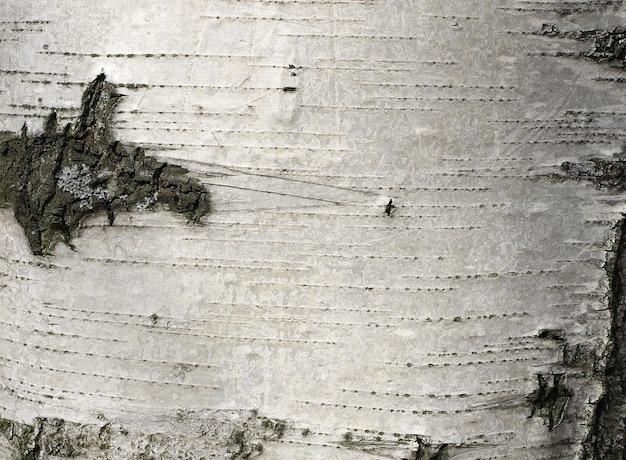This detailed close-up color photograph captures the textured trunk of a weathered birch tree. The prominent white bark is accentuated by distinctive black horizontal striations. In the upper left-hand corner, a break in the white bark reveals patches of gray bark, marbled with black cracks, and flecked with light green lichen. Similar gray and black cracked bark can be seen in the lower right-hand corner, also adorned with lichen. The intricate patterns and weathered appearance of the bark add depth and character to the image, highlighting the tree's natural beauty and resilience.